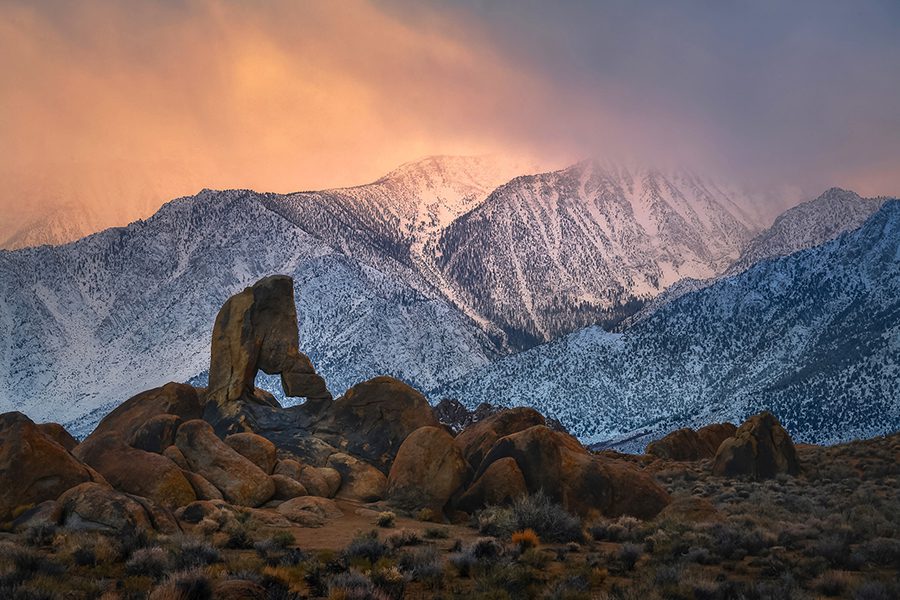The photograph captures a serene and relaxing landscape, likely taken during sunrise or sunset. The foreground is dominated by an assortment of brown dirt and stones of varying sizes, including larger boulders and smaller black stones. Scattered among the stones are patches of small grass. As the eye moves toward the middle of the image, you encounter a region filled with even larger boulder-sized stones. In the distance, a snow-covered mountain range stretches halfway across the image, its ridge line partially obscured by a haze of mist or smoke. The sky above is predominantly gray, except for the top left corner, which is tinged with orange-yellow hues from the sun attempting to break through the clouds, contrasted by darker blue tones on the right. The overall scene exudes tranquility, devoid of any human presence.